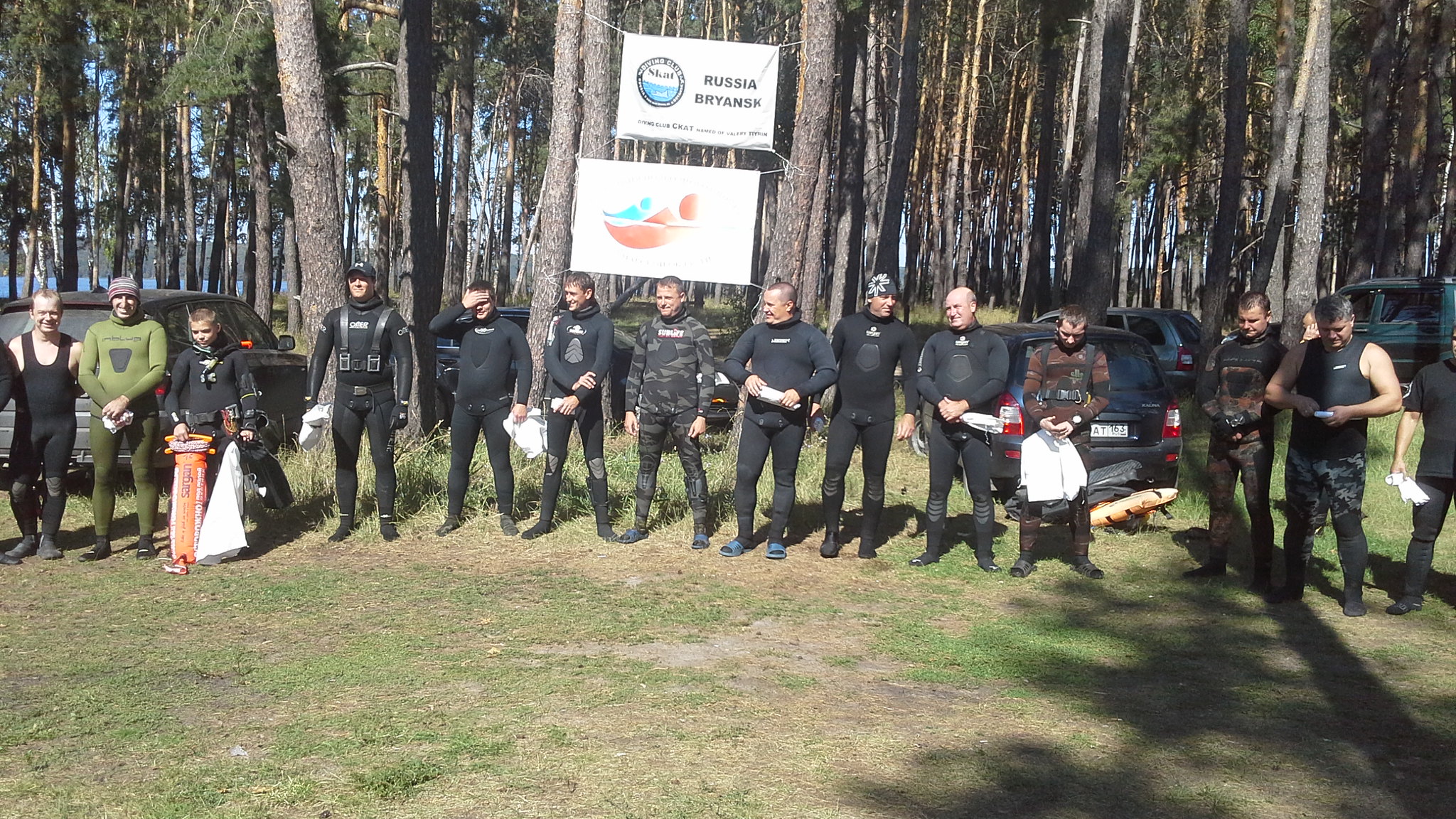In the photograph, a group of men is lined up in front of a dense forest backdrop, characterized by tall trees extending beyond the frame. The ground beneath them features a mix of dead and living grass. The men are primarily dressed in black attire that resembles wetsuits, with some variation including green tank tops and camouflage, as well as individuals both with and without sleeves. They are positioned in an organized, attentive stance, some smiling at each other.

Above their heads is a prominent banner that reads "Russia Bryansk," flanked by another sign displaying imagery suggestive of aquatic activities and the words "diving club Scott." Additional white signs with indecipherable text hang from the trees. Behind the men, cars are parked, further enhancing the outdoor setting. The overall scene suggests a formal or semi-formal gathering, possibly related to a diving club or similar organization.